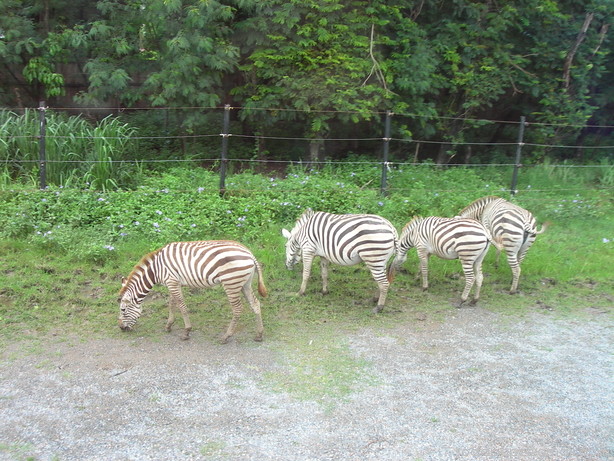This photograph features four zebras grazing on lush green grass near a rail fence composed of three wires strung between black metal posts. All the zebras are standing side by side with their heads down, focusing intently on the grass beneath them. The lower portion of the image shows a gravelly, grey ground with sparse patches of grass, transitioning to a more verdant middle section where the zebras are grazing. Small flower bushes with white blossoms are scattered near the fence. Behind the fence, a dense tree line of various types forms the backdrop, emphasizing a divide between the zebras' enclosure and the wild, forested landscape beyond.